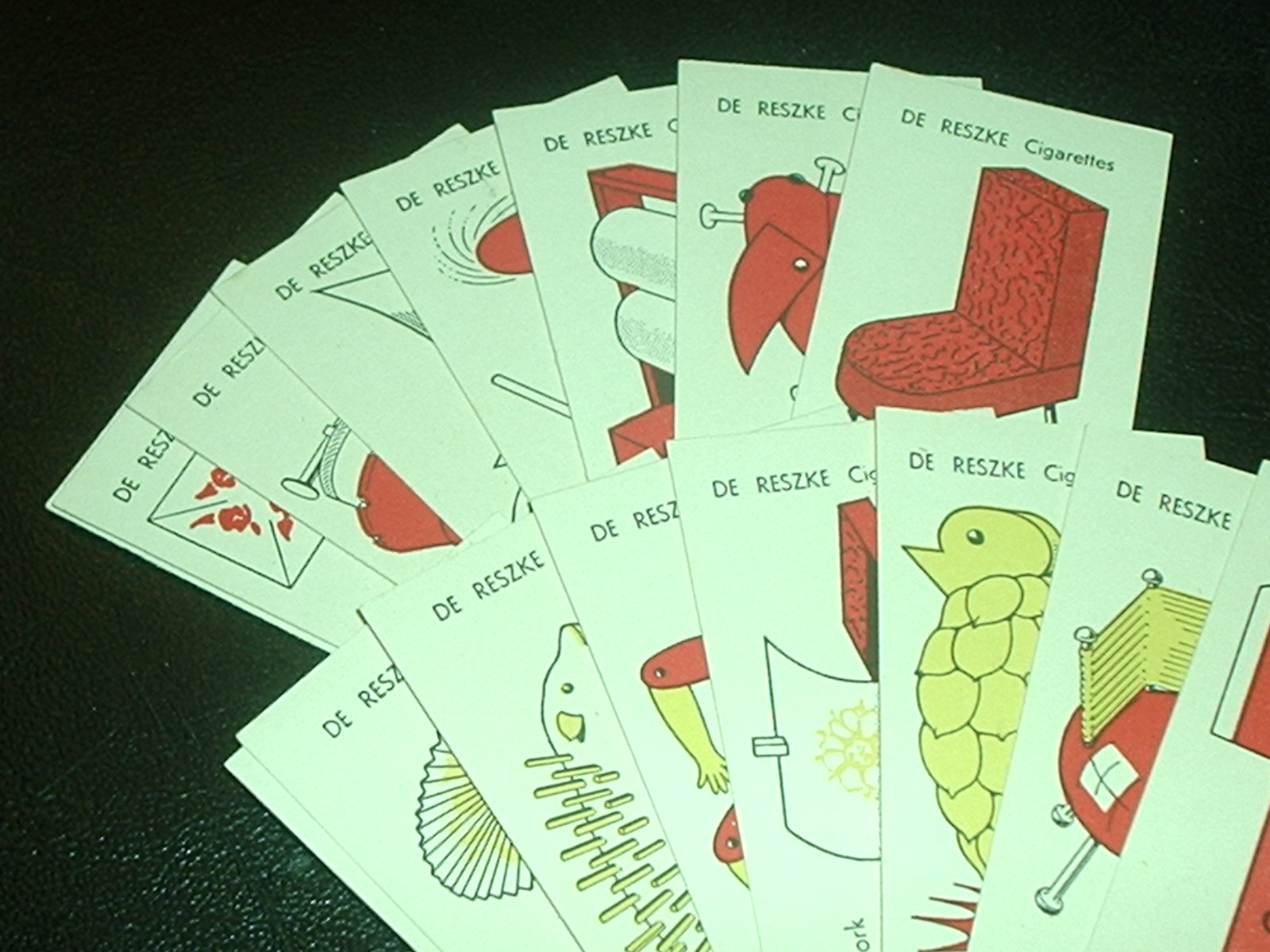This photograph captures an array of flashcards spread across a table, each featuring different images and words. The cards are predominantly white and adorned with cartoon-like illustrations in red and yellow hues. While most of the cards showcase words in a language other than English, one prominently displays the English word "cigarettes." Another card partially visible includes the word "D-E R-E-S-Z-K-E," which appears to be from a different language. The visible illustrations depict a variety of subjects, including what seems to be a chair, a bird, and possibly a puppet or a jointed toy. The cards' backgrounds contrast starkly with the black tabletop, making the colorful images and text stand out vividly.